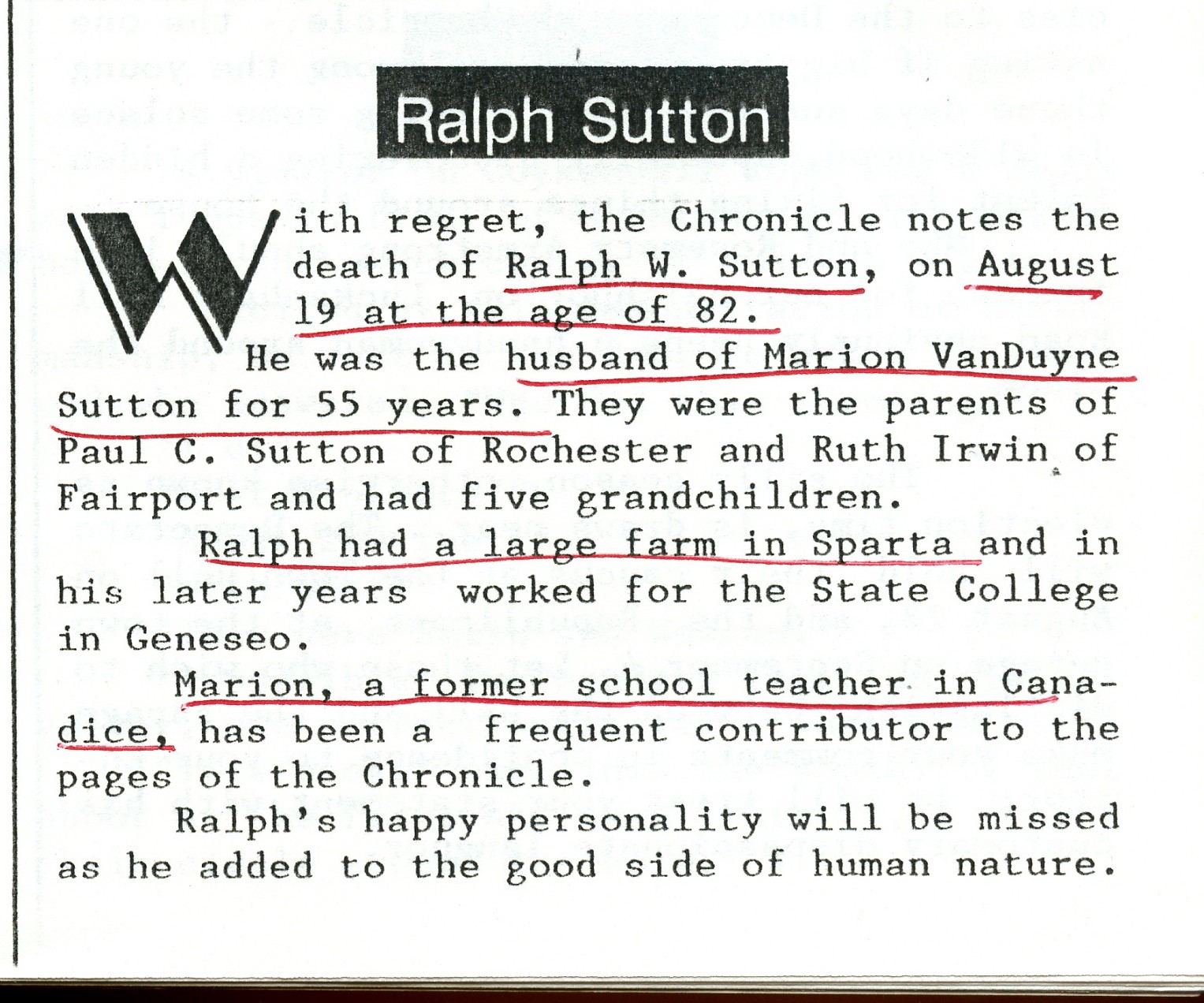This image shows a printed announcement of Ralph W. Sutton's obituary. The top of the page features a black rectangular box with "Ralph Sutton" written in bold white letters. Below, a large initial "W" introduces the text, "With regret, the Chronicle notes the death of Ralph W. Sutton on August 19th at the age of 82," with "Ralph W. Sutton" and the date "August 19th at the age of 82" underlined in red. Ralph was the husband of Marion Van Duane Sutton for 55 years, a detail also underlined in red. The couple had two children: Paul C. Sutton of Rochester and Ruth Irwin of Fairport, along with five grandchildren. Ralph owned a large farm in Sparta, a fact highlighted by a red underline, and in his later years, he worked for the State College in Geneseo. Marion, a former schoolteacher in Canadies (underlined in red), was a frequent contributor to the Chronicle. The announcement concludes by noting Ralph’s positive contributions to human nature, emphasizing that his happy personality will be greatly missed. The page is bordered by thin black lines on the left side and at the bottom, further framing this heartfelt tribute.